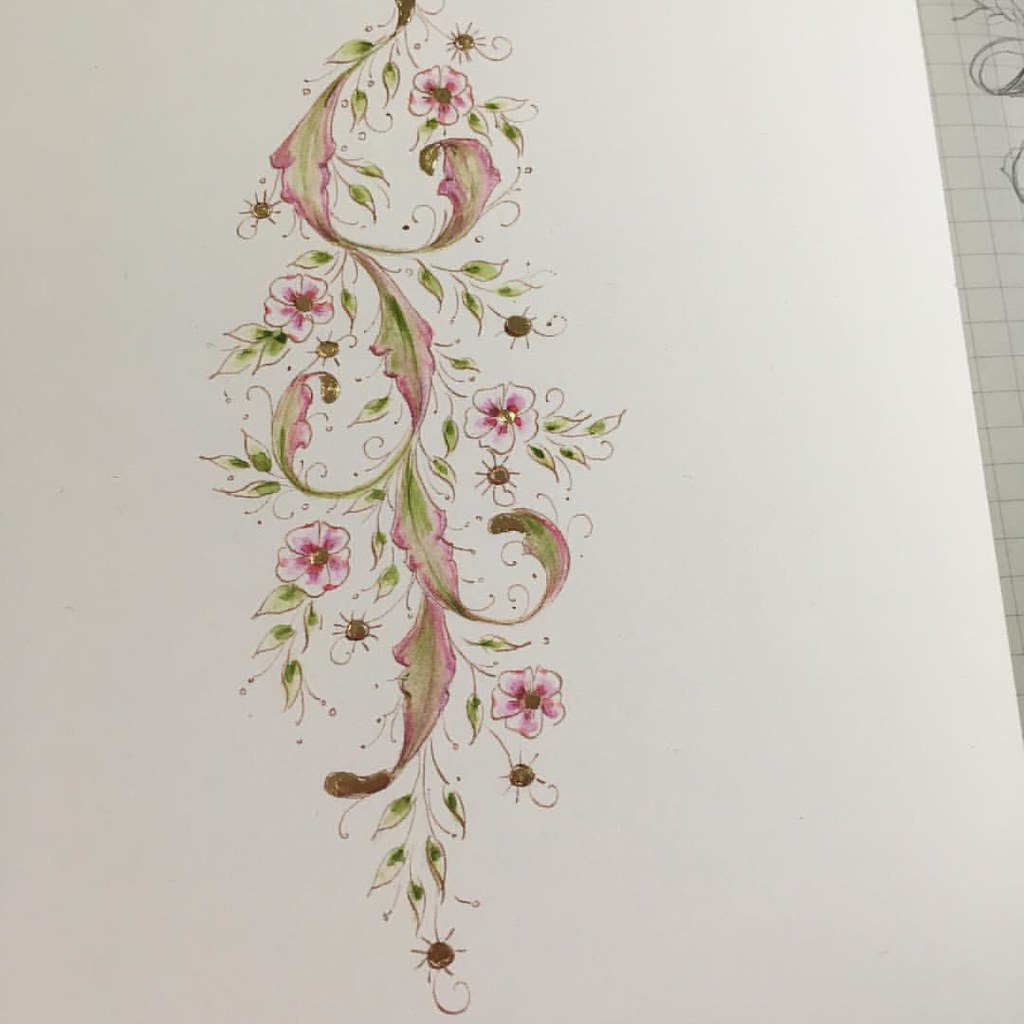This is a detailed, calligraphic-style illustration on a white piece of drawing paper. The artwork features a long, slender, acanthus-like vine running vertically down the center of the page, somewhat reminiscent of a modern William Morris wallpaper design. The image is created with what appears to be watercolor or colored ink, featuring predominantly pink and green hues. The vine is adorned with stylized leaves that are green with pink edges, along with various small flowers and buds. Some of the flowers are purple with white-tipped petals. The tendrils of the vine extend to the sides, displaying a variety of floral elements, including buds and seed pods. On the right edge of the drawing, there's a glimpse of kid's graph paper with some pencil doodles, enhancing the handcrafted feel of the piece. The composition is both intricate and delicate, blending floral motifs and botanical details in a visually appealing manner.